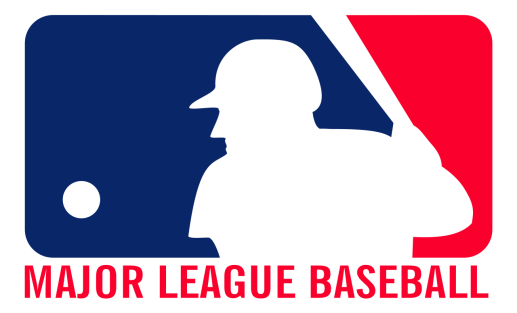The image displays the iconic logo for Major League Baseball (MLB), which features a rectangle with rounded corners set against a white background. The left portion of the logo is filled with a deep blue color, while the right side is a vibrant, fire truck red. In the lower left corner of the blue section, there's a small white circle, symbolizing a baseball. Dominating the center to the right side, bridging the transition from blue to red, is a white silhouette of a baseball player wearing a cap. The player is poised to hit, with a raised bat ready to strike the ball. The figure is depicted in a way that the back faces the viewer, seemingly looking out towards the pitcher's mound. Below the rectangle, in bold red uppercase letters, the words "MAJOR LEAGUE BASEBALL" are prominently displayed. This digitally designed logo is a universally recognized symbol of the MLB.